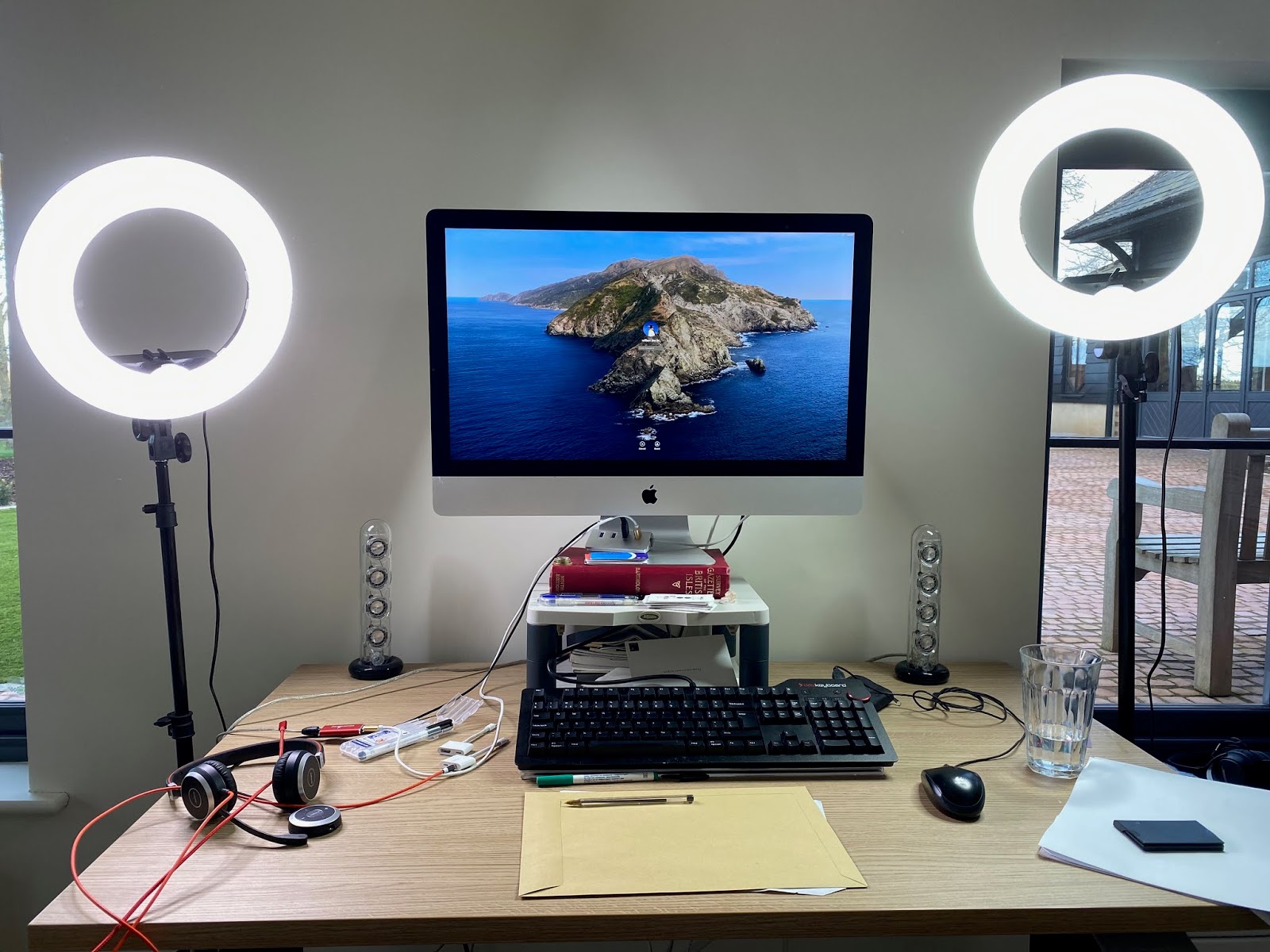The image depicts a modern workspace set against a white wall with subtle natural light coming from a window to the left, where some grass is visible, and another window to the right with a white chair on a brick patio outside. Predominantly in the center is a light brown desk, cluttered yet orderly, suggesting the space is actively used, likely by a content creator or YouTube influencer. A screen, possibly part of an all-in-one Apple computer or a solely wall-mounted display, showcases an image of a rocky island emerging from a blue ocean. The screen is enhanced by two ring lights with circular white surfaces and black support rods, framing the workspace for optimal lighting.

On the desk, a variety of items are neatly arranged: a black mechanical keyboard centered with a brown notebook and pen directly in front. To the left is a pair of gaming headphones with an orange cable, laying beside what appears to be a listening or recording device stacked on a stand. The right side houses a black computer mouse and a clear glass filled one-quarter with water, placed near a weight resting atop a white stack of papers. Two tall, clear plastic Apple speakers with stacked components and black bases flank the monitor, supported by numerous cables and possibly connected to the computer setup via a rudimentary stand.

To accentuate the aesthetic and functional sophistication, two modern ring lights flank the setup, aligning to provide perfect illumination for content creation, reinforcing the impression of a workspace designed for high-quality video recording and streaming. The desk also features some decorative clear circles encased in glass on either side of the keyboard, adding to the personalized and professional feel of the setup.